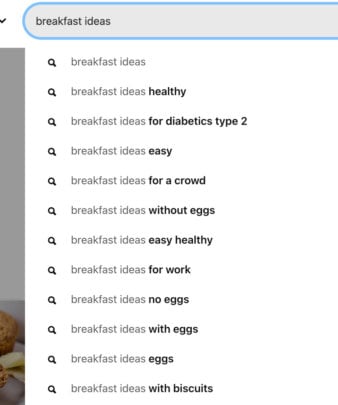The image displays a search bar prominently outlined in blue, with the phrase "breakfast ideas" typed into it. Below the search bar, there is an extensive drop-down menu showcasing a list of approximately twelve suggestions. Each entry in the list features a black, slanted magnifying glass icon on the left, followed by bold text indicating various types of breakfast ideas. The entries in the list appear as follows:

1. Breakfast ideas
2. Breakfast ideas healthy
3. Breakfast ideas for diabetics type 2
4. Breakfast ideas easy
5. Breakfast ideas for a crowd
6. Breakfast ideas without eggs
7. Breakfast ideas easy healthy
8. Breakfast ideas for work
9. Breakfast ideas no eggs
10. Breakfast ideas with eggs
11. Breakfast ideas eggs
12. Breakfast ideas with biscuits

The drop-down menu itself is set against a clean, white background. Partially visible behind this drop-down menu is a webpage with imagery, likely food-related, but much of it is obscured and its full content is indiscernible.